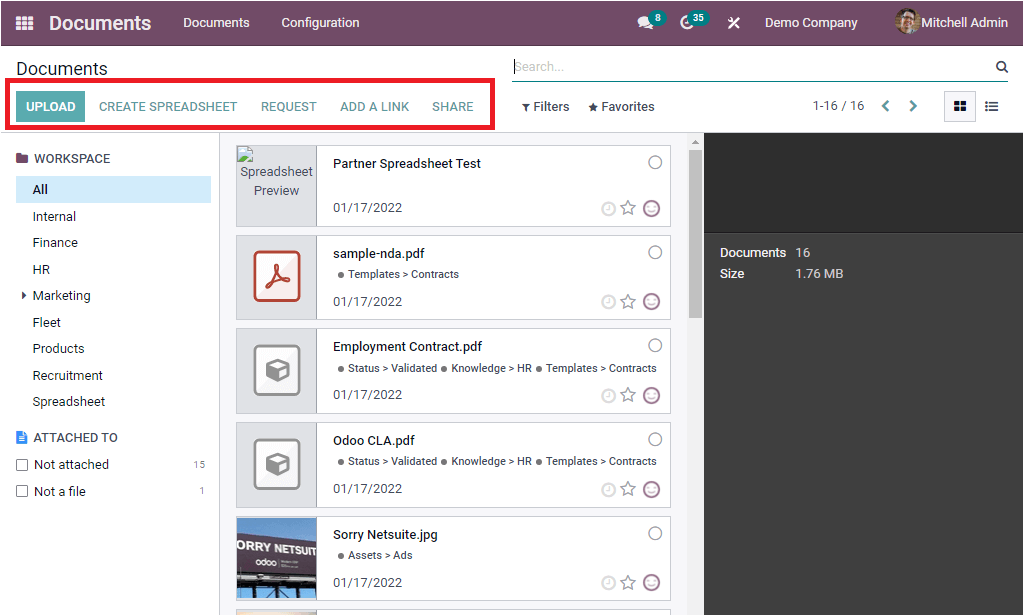This screenshot showcases a computer screen displaying a document management interface. The prominent section highlights a red rectangular box under a "Documents" heading. Within this box, there are options, including "Upload" (highlighted in green), "Create Spreadsheet," "Request," "Add Link," and "Share." A folder labeled "Workspace" appears below, with subcategories such as "All," "Internal," "Finance," and "HR." An arrow next to "Workspace" suggests expandable options, with additional subfolders like "Marketing," "Fleet," "Products," "Recruitment," and "Spreadsheet."

Next to these, icons indicate file status: one file is attached with a file icon, fifteen are marked as "Not Attached," and one falls under "Not a File."

In the central part of the screen, there are five specific files listed:
1. Partner Spreadsheet Test
2. Sample NDA (PDF format)
3. Employee Contact (PDF format)
4. Odole CLA (PDF format)
5. Sorry Nate Suite (JPEG format).

On the left side of the image, a black panel indicates "Document 16" with a file size of 1.76 megabytes. At the top of the screen, several icons are visible: a message icon indicating eight messages, an additional icon showing thirty-five (possibly notifications), a Help Tool, and elements labeled "Demo Company" and "Michael Admin."